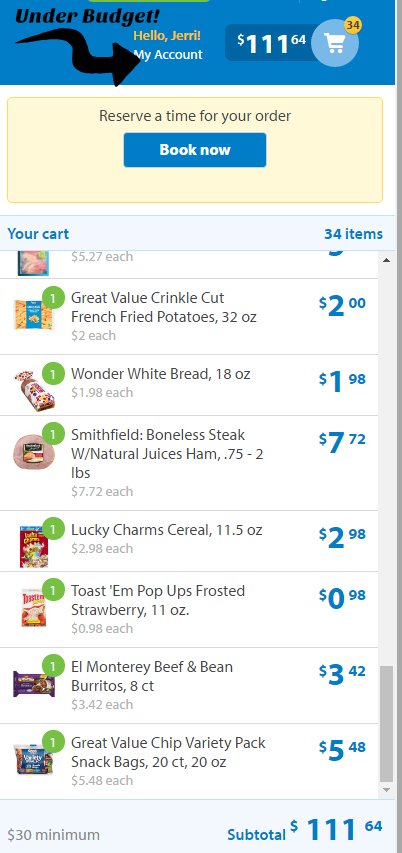The image depicts a person navigating an online grocery shopping app on a cell phone. The proportions and layout suggest it's a vertical rectangle, typical of a smartphone screen. The top area is obscured, but it hints at essential cell phone interface details such as signal bars or clock.

The screen's top section features a blue bar displaying "Under Budget" with a small black swirly arrow beside it. Below this, there's a greeting text "Hello Jerry," with the name spelled "J-E-R-R-I," followed by a link to "my account." To the far right, a shopping cart icon indicates there are 34 items currently in the cart.

The main section reveals more detailed information about the shopping cart, totaling an estimated $111.64 worth of items. A prominent yellow banner urges the user to "Reserve a time for your order," with a blue "book now" button available for scheduling.

The list of items in the cart is detailed, featuring product images, quantities, and prices. For example, there's a listing for Great Value Crinkle-Cut French Fried Potatoes, 32 ounces priced at $2.00, along with an accompanying icon and a green circle indicating the quantity. Another item is Wonder White Bread, 18 ounces for $1.98, followed by Smithfield Boneless Ham with Natural Juices, priced at $7.72 per 0.75-2 pounds.

This image vividly captures the process of someone actively engaged in ordering groceries online, efficiently selecting and managing their preferred items.